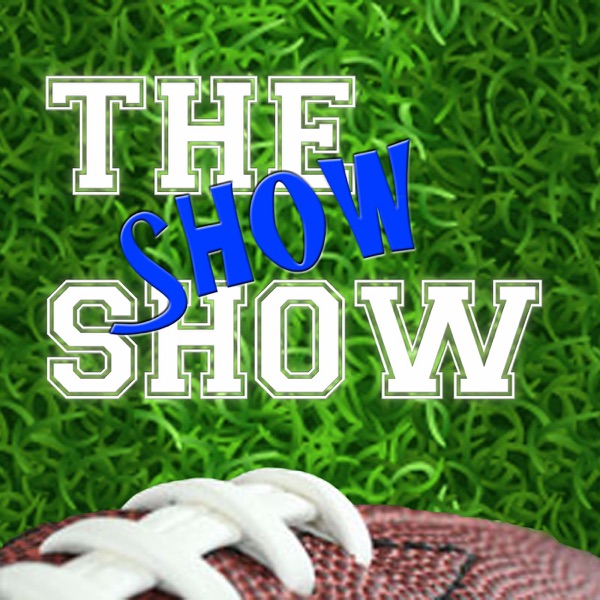The image features a predominantly green background of artificial turf, occupying about 80-85% of the frame, giving the impression of looking down at a grassy field. Central to the composition is bold, tri-layered text that reads "THE SHOW SHOW." The first "SHOW" is in bold white lettering, the second diagonally across in blue, and the final "SHOW" again in white. At the bottom of the image, partially cut off but clearly visible, is a brown football with prominent white laces, detailed and up close. The setting is bright, suggesting natural light, and the overall style hints at a promotional graphic for a web show or TV show. The colors in the image include various shades of green, white, gray, blue, and brown.